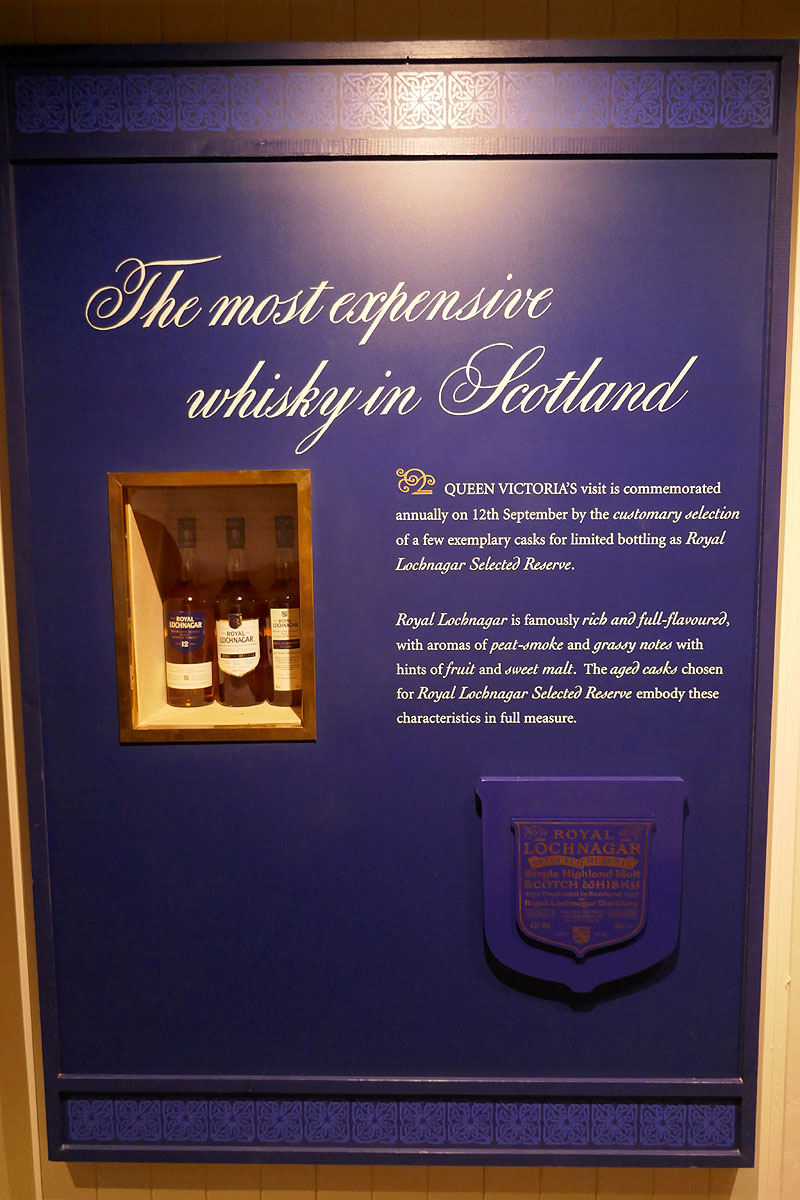This real-world photograph features an elaborate display highlighting an exclusive whiskey brand. Centered on a large blue platform, a smaller rectangular cutout towards the left side holds three carefully placed bottles of Royal Lochnagar whiskey. The surrounding blue board prominently features a detailed write-up in white letters explaining the significance of the whiskey. The text reads: "The most expensive whiskey in Scotland. Queen Victoria's visit is commemorated annually on 12th September by the customary selection of a few exemplary casks for limited bottling as Royal Lochnagar Selected Reserve. Royal Lochnagar is famously rich and full-flavoured, with aromas of peat smoke and grassy notes with hints of fruit and sweet malt. The aged casks chosen for Royal Lochnagar Selected Reserve embody these characteristics in full measure." Positioned at the bottom right of this text, a company logo appears, adding to the luxurious presentation.